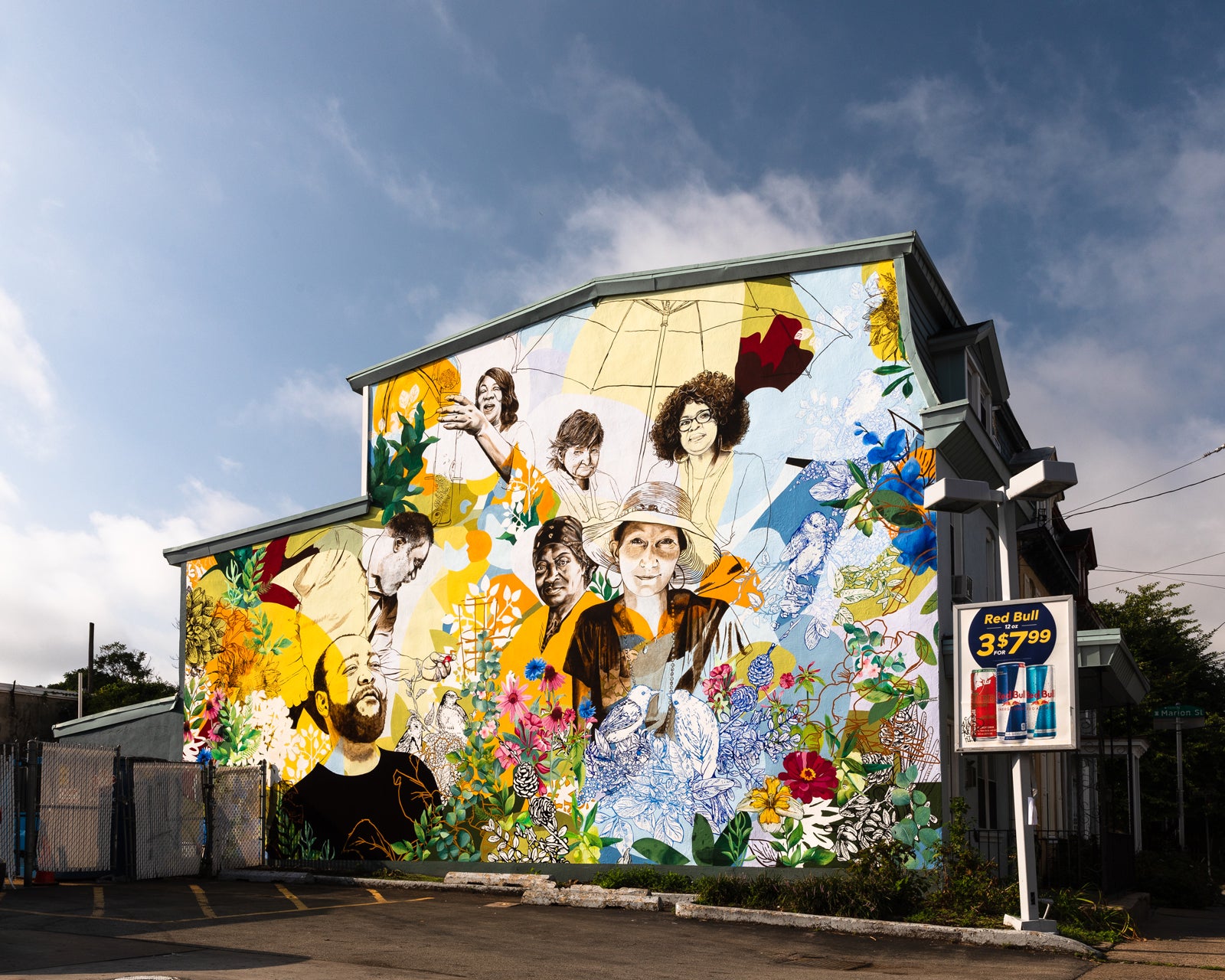This is an outdoor photograph depicting a large, rectangular mural on the side of a two-story high building, captured during the daytime. The sky is a cloudy blue backdrop above the structure. The mural itself features detailed drawings of seven people, a mix of men and women, surrounded by colorful birds and an array of flowers. On the left-hand side of the mural, a man with a mustache and beard, dressed in a black shirt, is portrayed gazing to the right. Above him, another man is illustrated looking downward, holding a red object in his hand. To the right of the building, a sign advertising "Red Bull, 3 for $7.99" is visible. The lower part of the image reveals a parking area on the left, bordered by metal gates with white plastic serving as a privacy screen. The artwork is the centerpiece, bringing vibrancy and character to the otherwise utilitarian side of the building.